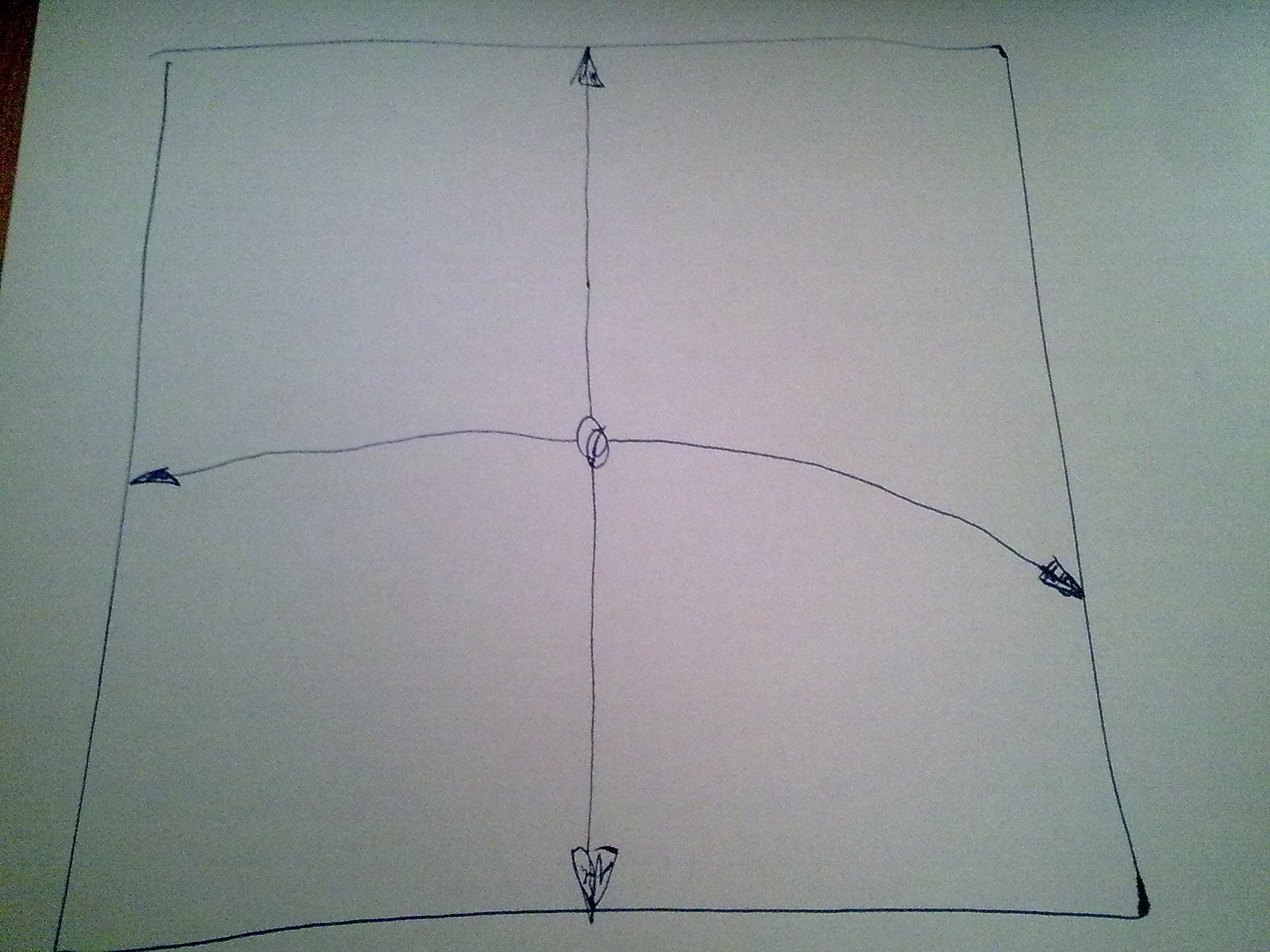The image features a sheet of printer paper, partially resting on a dark brown wooden table, only a small portion of which is visible on the left-hand side of the frame. The paper contains a hand-drawn blue ink diagram centered around a roughly sketched square. In the middle of this square is a hastily scribbled circle, from which four somewhat wavy lines extend outward in the cardinal directions: up, down, left, and right. The rightward line notably veers slightly downward. At the terminal point of each line is a heavily drawn triangle, appearing as if they were repeatedly traced to achieve their intended form, resulting in a dense and somewhat irregular outline. The entire drawing gives an impression of spontaneity and imperfect symmetry, adding a human touch to the simple geometric design.